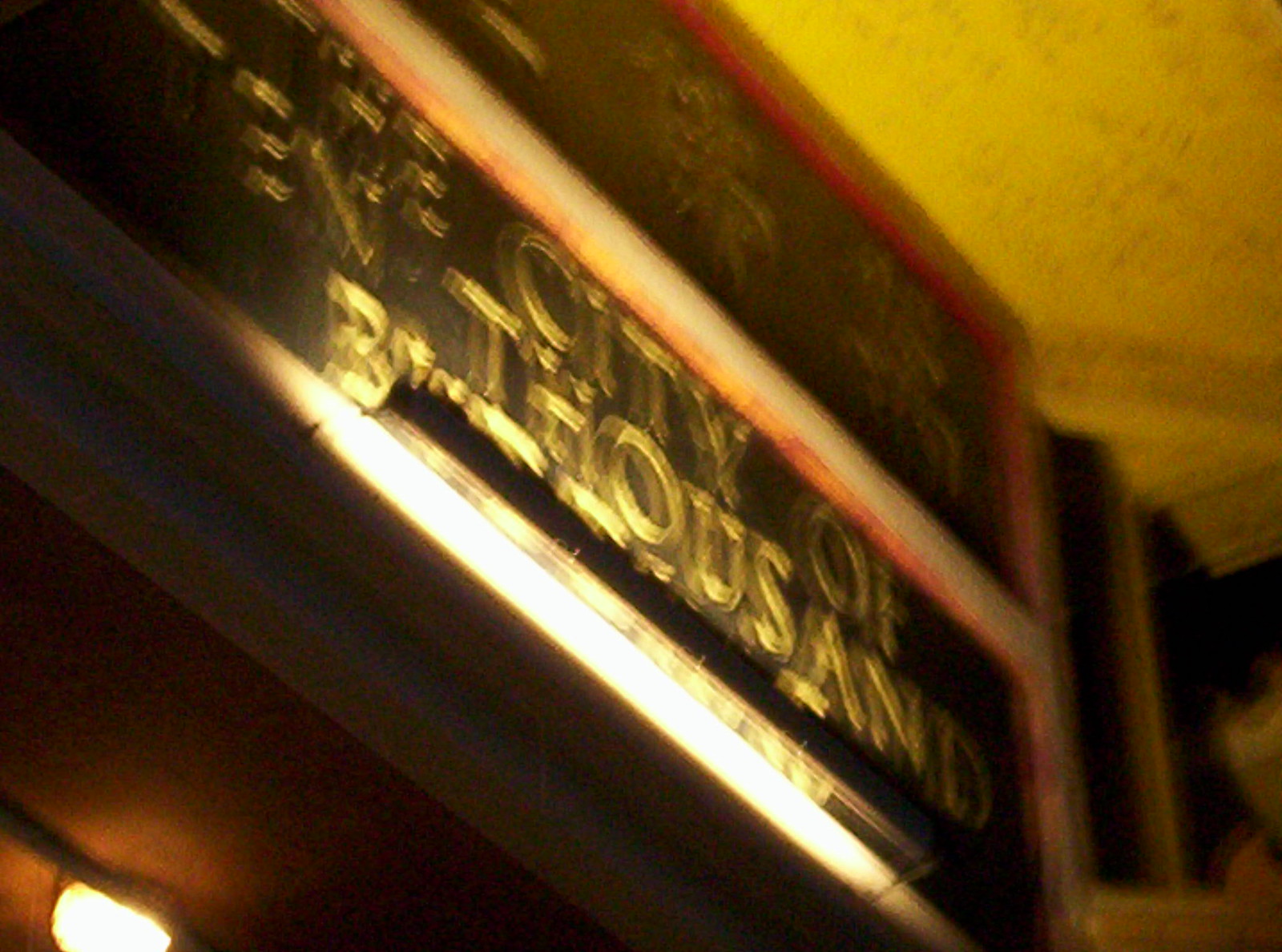This image is a very blurry photograph taken in low-light conditions, likely with some motion blur. The primary focus is a sign above a doorway, which has a black background with raised gold letters. Part of the sign reads "City of Thousand," though additional words are cut off and unreadable. There is an additional sign above this one with raised characters in Chinese script, suggesting the location might be a Chinese restaurant or shop. To the top right of the image, there is a ceiling that appears to be a stone color but has a yellowish tint due to a reflected yellow light. The bottom left of the image shows a darkened area, possibly the underside of the sign, with a circular yellow light. The overall ambiance suggests an urban setting, potentially at night, adding to the difficulty in capturing a clear image.